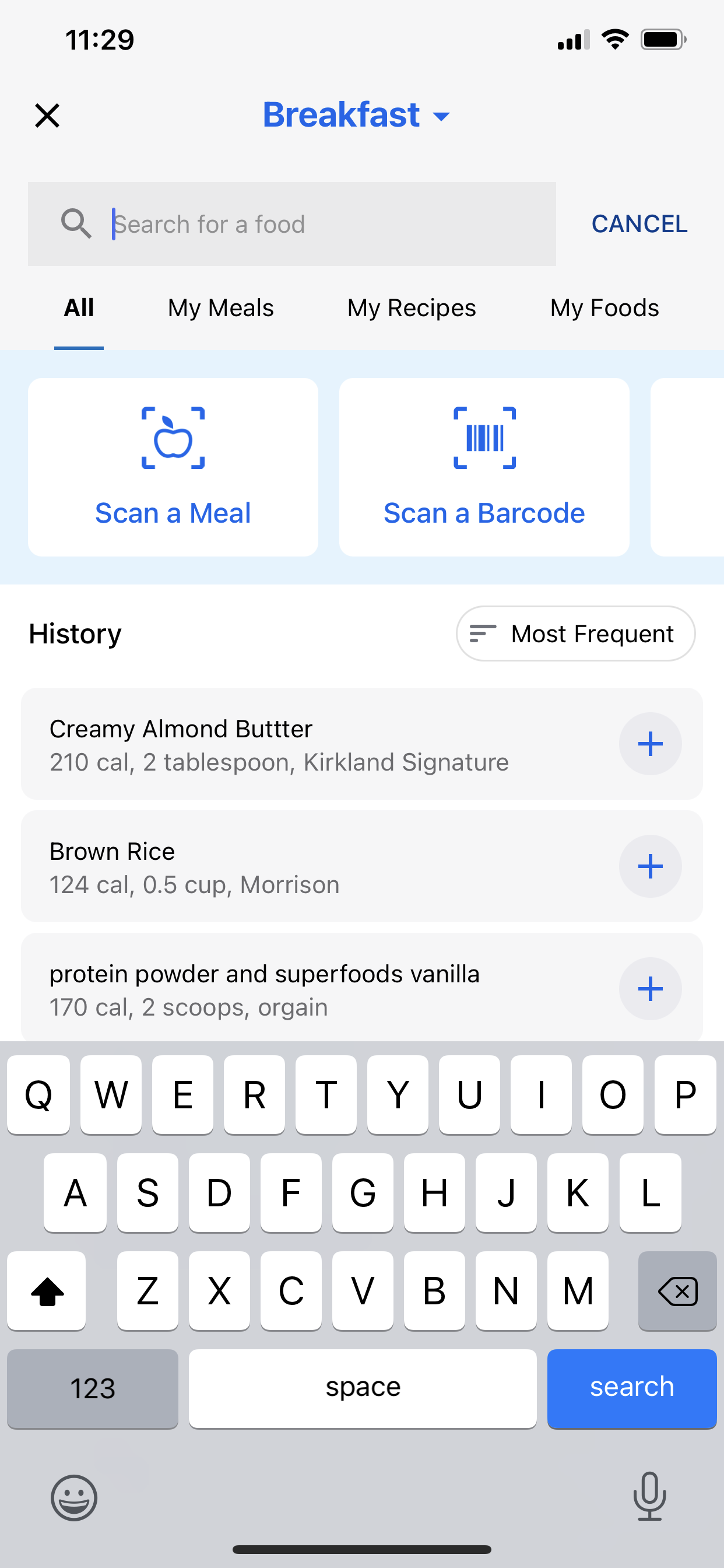This detailed screenshot captures a phone interface displaying a nutritional tracking app. At the top of the phone screen, the time reads 11:29, with icons indicating a full battery, full Wi-Fi signal, and three-quarters network coverage. The app is currently on the "Breakfast" section, prominently displayed at the top alongside a drop-down menu icon and an 'X' button for closing the section.

Below the header, there is a search bar with the placeholder text "Search for food." Under it are menu options labeled "All My Meals," "My Recipes," and "My Foods." The app provides two large rectangular buttons beneath the search bar labeled "Scan a Meal" and "Scan a Barcode," offering easy access for quick food logging.

Continuing down, the screen shows the user's food history sorted by most frequently consumed items. The first item listed is "Creamy Almond Butter," containing 210 calories per 2 tablespoons from the Kirkland Signature brand. The second item is "Brown Rice," with a calorie count of 124 per half-cup, from the Morrison brand. The third item is "Protein Powder, Superfoods, Vanilla," which has 170 calories per 2 scoops from the Orgain brand.

At the bottom of the screenshot, the phone's Apple QWERTY keyboard is visible, with keys in the classic layout: Q, W, E, R, T, Y, U, I, O, P on the first row.

This future-oriented, snapshot view takes us through a meticulous interface designed to track and manage food intake efficiently.